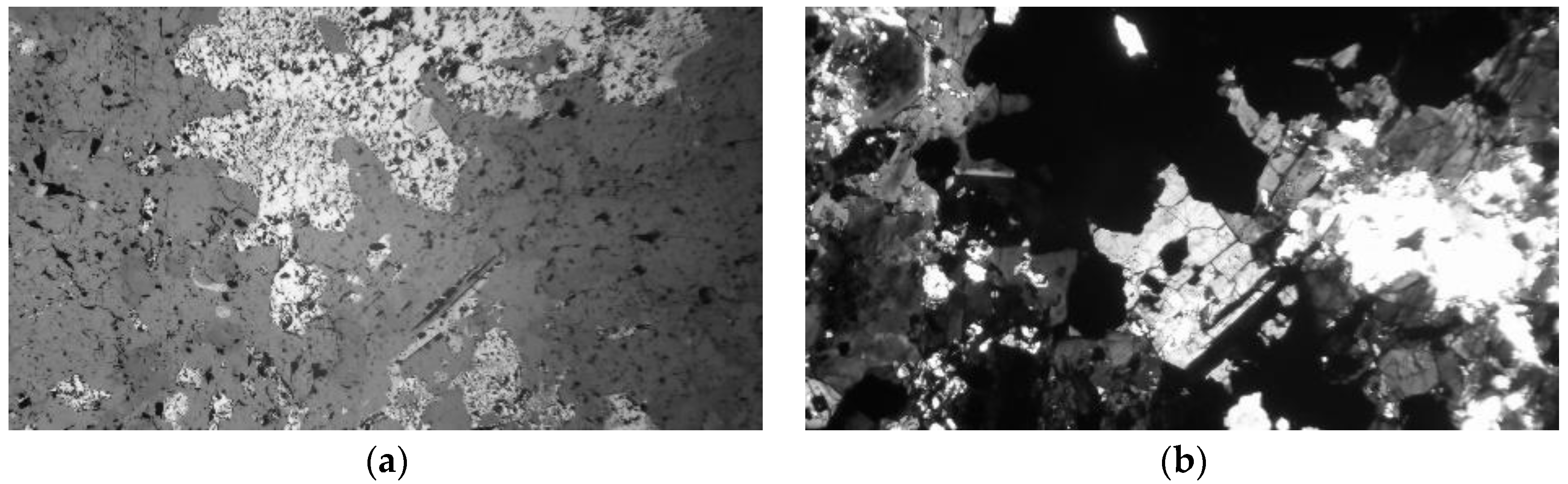The image displays two horizontally-aligned, black-and-white abstract rectangular images, labeled (a) on the left and (b) on the right. Both images could represent various interpretations, such as satellite views of landmasses, microscopic slides, or stone surfaces with varying textures and shades.

Image (a) shows a predominantly darker gray surface speckled with black marks, suggesting a worn, textured appearance similar to an old marble wall or stone surface. Its upper center features a whiter, edged area that stands out against the darker background, resembling a landmass viewed from above or an area of higher intensity on a spectroscopic slide.

Image (b) is characterized by a predominantly black background with irregular white and gray blotches. It appears even more abstract than image (a), featuring a few high-intensity white areas that contrast sharply with the black. Overall, image (b) has larger white splotches compared to the more evenly distributed speckling in image (a), giving it a more fragmented and varied appearance.

Together, these images offer different abstract representations, primarily highlighting a stark contrast in textures and intensity between the grayscale areas.